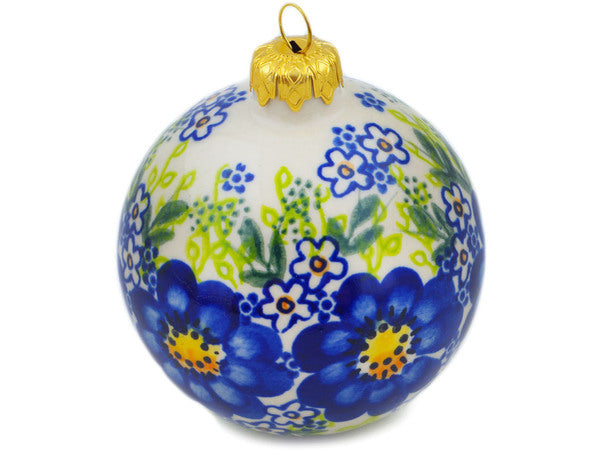The image features a detailed photograph of a Christmas bauble ornament set against a stark white background. The bauble itself is predominantly white and appears to be hand-painted, giving it a slightly opaque, yet mostly solid appearance. Central to its design are two large, intricate blue flowers prominently displayed in the middle. These flowers feature dark blue edges with lighter blue centers, which are highlighted by vibrant yellow and orange centers adorned with dark blue spots.

Surrounding these large blooms are smaller white and blue flowers—two located at the top and two at the bottom of the ornament. The floral design is complemented by painted green leaves, which vary in shade from dark green to lime green, adding depth and variety to the decoration. Additionally, small blue dots are scattered among the greenery, representing tiny flower buds.

The ornament is topped with a gold hook and ring attachment, making it ready to be hung on a Christmas tree. This combination of colors and details creates a richly decorated and visually appealing Christmas bauble.